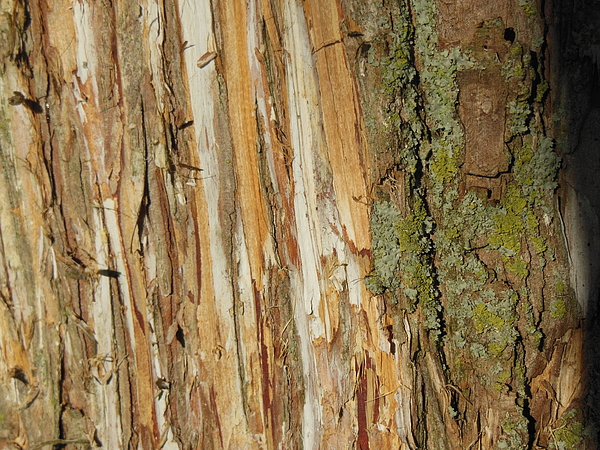This close-up, square photograph, taken at night, features a tree with significant bark damage. The tree's trunk is brightly lit against the dark sky, illuminating the details vividly. Approximately two-thirds of the left side of the tree has been stripped of its dark brown bark, revealing an intricate mosaic of the tree's inner wood in shades of white, light tan, brown, and orange, indicating recent exposure, possibly due to chopping or accidental damage such as a car collision. The remaining bark on the tree features thick patches of lime-green and turquoise-colored lichen or mold, particularly concentrated on the right-hand side of the trunk. The detailed texture of the exposed wood contrasts sharply with the mottled green and turquoise lichen that covers the intact bark. No people, text, or other objects are present in the image, focusing solely on the intricate, multicolored patterns of the damaged tree trunk.